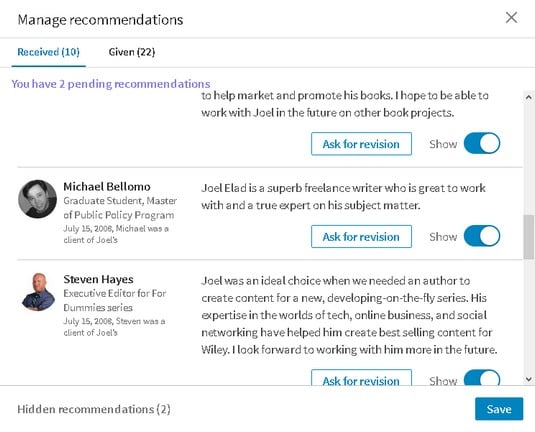The image displays a section of a website interface dedicated to managing recommendations. The top of the interface features the heading "Manage Recommendations." Below this heading are two tabs: "Receive" and "Given," with numerical indicators in parentheses stating "(10)" and "(22)" respectively. A notification follows, indicating that there are "2 pending recommendations."

To the right side of the interface, part of a text appears to be crossed out, with a visible remaining portion stating: "To help market and promote his books, I hope to be able to work with Joel in the future and on other book projects." The remaining part of the image appears to show descriptions of two other individuals, though specific details are not provided in the current view.